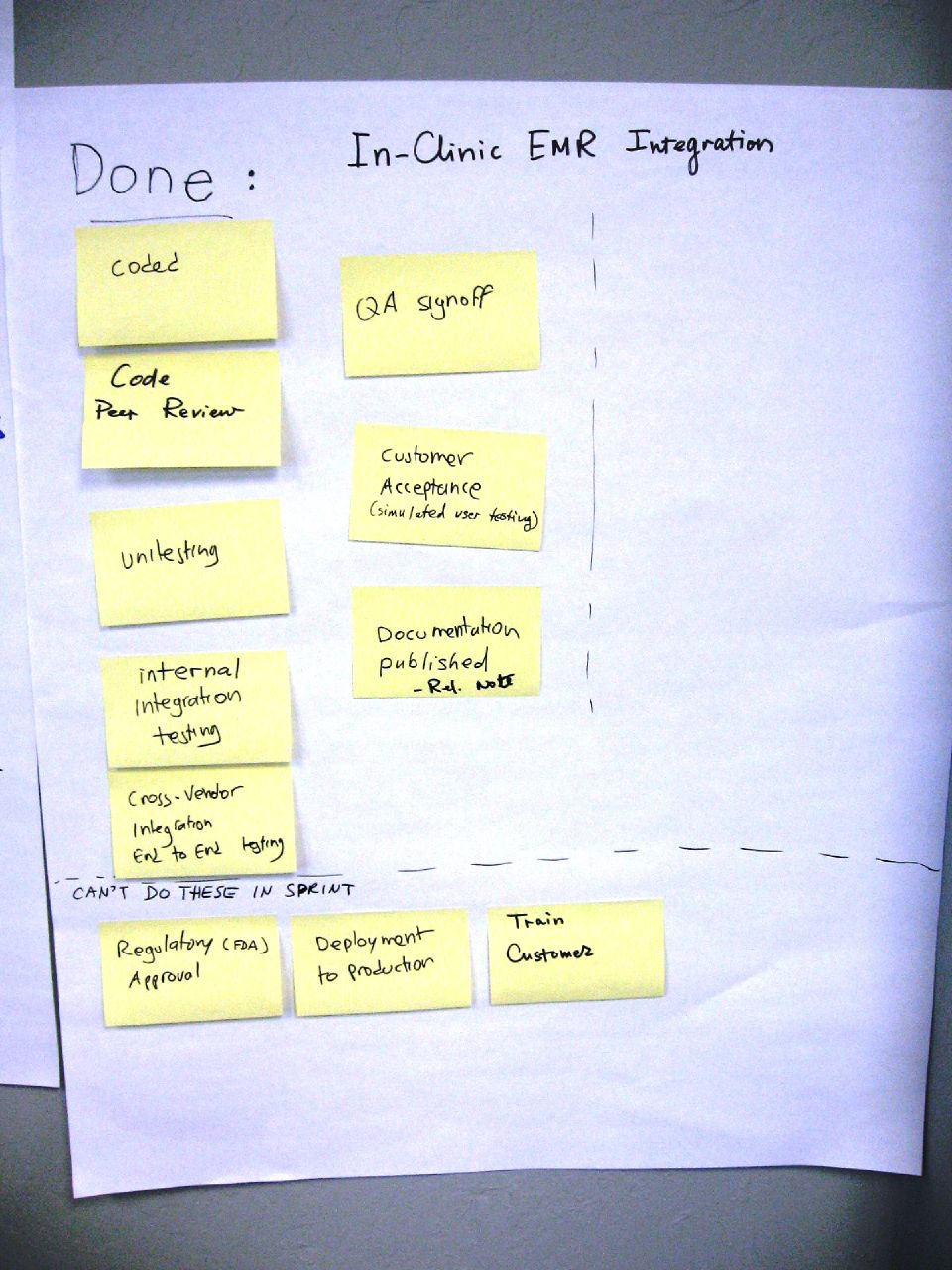The image depicts a handmade chart drawn on a crinkled white piece of paper, slightly tinged with blue. The chart is divided into three main sections using columns of yellow post-it notes. At the top, the title "In Clinic EMR Integration" is written in black thin magic marker, followed by a subheading that reads "Done." Below this subheading, a detailed list of tasks is organized on individual post-it notes, including "Coded," "Code Peer Review," "Unit Testing," "Internal Integration Testing," "Cross Vendor End-to-End Testing," "QA Sign-Off," "Customer Acceptance," "Simulated User Testing," and "Documentation Published." The section also mentions "Rel Note." 

A dotted line separates this segment from the next section, titled "Can't Do These in Sprint," which contains post-it notes with tasks like "Regulatory Approval," "Deployment to Production," and "Train Customer." The arrangement of post-it notes includes two main columns and a third column below them, leaving a significant portion of the right side of the sheet blank. The paper's edges are slightly worn and curled, giving a handmade and utilitarian feel to the chart.